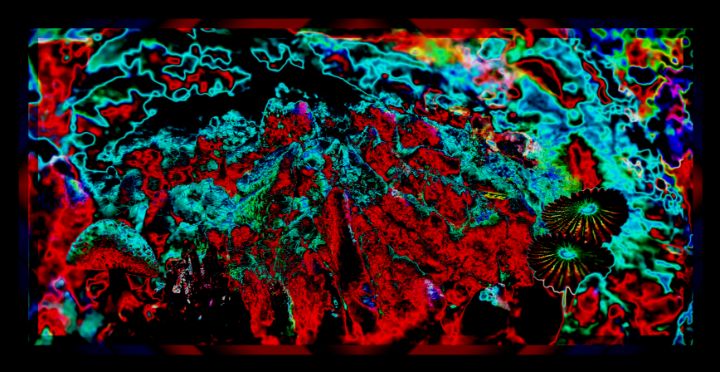The image is a long, rectangular black background reminiscent of a blacklight poster from the 60s hippie era, imbued with a highly psychedelic and abstract pattern. It's an explosion of vibrant, fluorescent colors including patches of bright red, teal, blue, yellow, green, purple, and orange, creating a high-contrast, kaleidoscopic effect. The scene evokes the appearance of thermal imaging, displaying organic, irregular shapes that resemble the forest floor strewn with random debris and rocks, as well as coral formations. The foreground features discernible shapes, including two small flowers with many petals around a central circle in the bottom right corner, standing out amongst the scattered, high-contrast colors. This visually intense and detailed composition feels like an image enhanced with filters and tweaked contrast, designed to evoke a sense of psychedelic wonder.